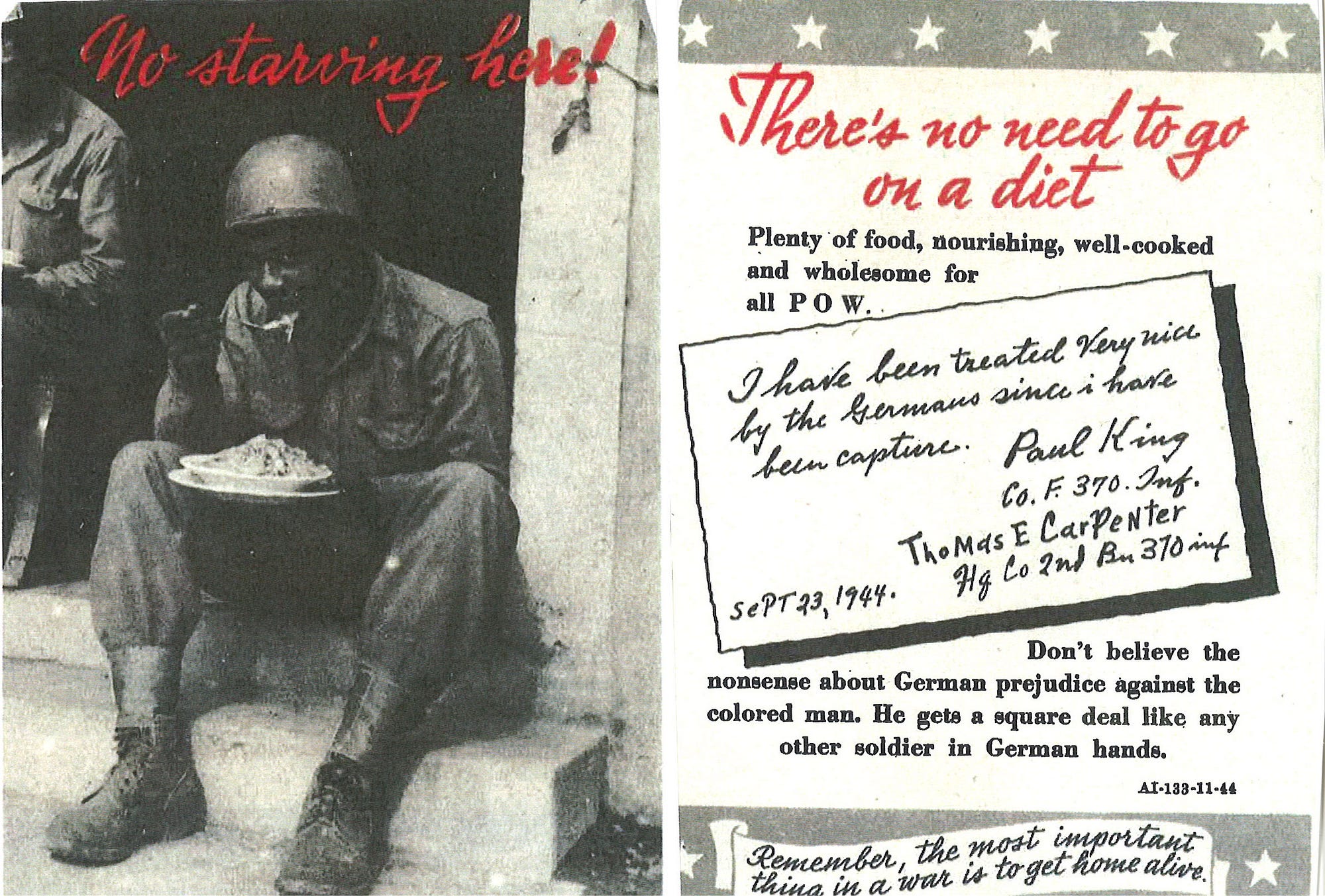The image appears to be an old propaganda postcard from World War II, designed by the German Nazis. It is rectangular, approximately six inches wide and four inches high, depicting a black and white photograph on its left side. The photograph features a man of African descent, dressed in a military uniform and wearing a bucket hat, sitting on some steps. He is holding a plate of food, about to take a bite. Above the photo, in red cursive text, it states, "No Starving Here."

The right side of the postcard is filled with various textual elements. At the top in red text, it reads, "There's No Need to Go on a Diet." Below this, black text proclaims, "Plenty of Food, Nourishing, Well-Cooked, and Wholesome for All P.O.W.s." In the center of the right side is a tilted, postcard-like rectangle containing handwritten, cursive text that says, "I Have Been Treated Very Nice by the Germans Since I Have Been Captured," signed by Paul King, Company F, 370 Infantry, and Thomas E. Carpenter, H.D. Company, 2nd Battalion, 370 Infantry. It is dated September 23, 1944. 

Further down, black text insists, "Don't Believe the Nonsense About German Prejudice Against the Colored Man. He Gets a Square Deal Like Any Other Soldier in German Hands." At the bottom of the postcard is a white ribbon-like banner with black cursive text that reads, "Remember, the Most Important Thing in a War is to Get Home Alive."

The postcard is evidently meant to convey the message that prisoners of war, regardless of race, were well treated by the Germans, countering any claims of racial prejudice.